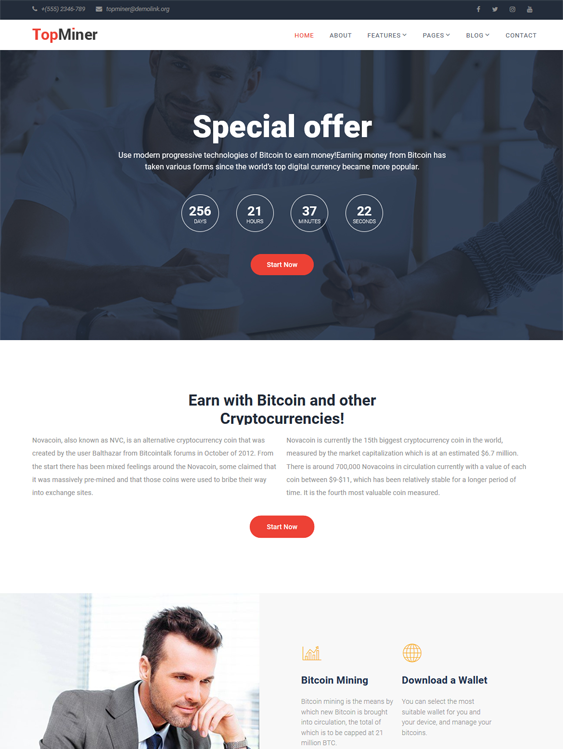Top Miner Special Offer: Harness Modern Progressive Technologies to Earn Bitcoin

Explore the innovative world of Bitcoin mining with Top Miner. Utilizing cutting-edge technologies, this platform provides users with various avenues to earn money through the world's leading digital currency. 

At the top of the page, you'll find navigation links including Home, About, Features, Pages, Blog, and Contact, along with a striking background image of three professionals engaged in a discussion in an office setting. This area features a dynamic countdown clock, currently displaying 256 days, 21 hours, 37 minutes, and 22 seconds. A prominent "Start Now" button invites immediate participation.

Scrolling down further, users are encouraged to earn with Bitcoin and other cryptocurrencies. The page introduces NovaCoin (NVC), an alternative cryptocurrency, and elaborates on its features. A secondary "Start Now" button offers another opportunity to dive in.

The next section includes a stock photo of a man at a desk, engrossed in his laptop, as additional information about mining processes and digital wallets is presented. The overall tone is corporate and professional, reflecting the seriousness and widespread interest in cryptocurrency mining.